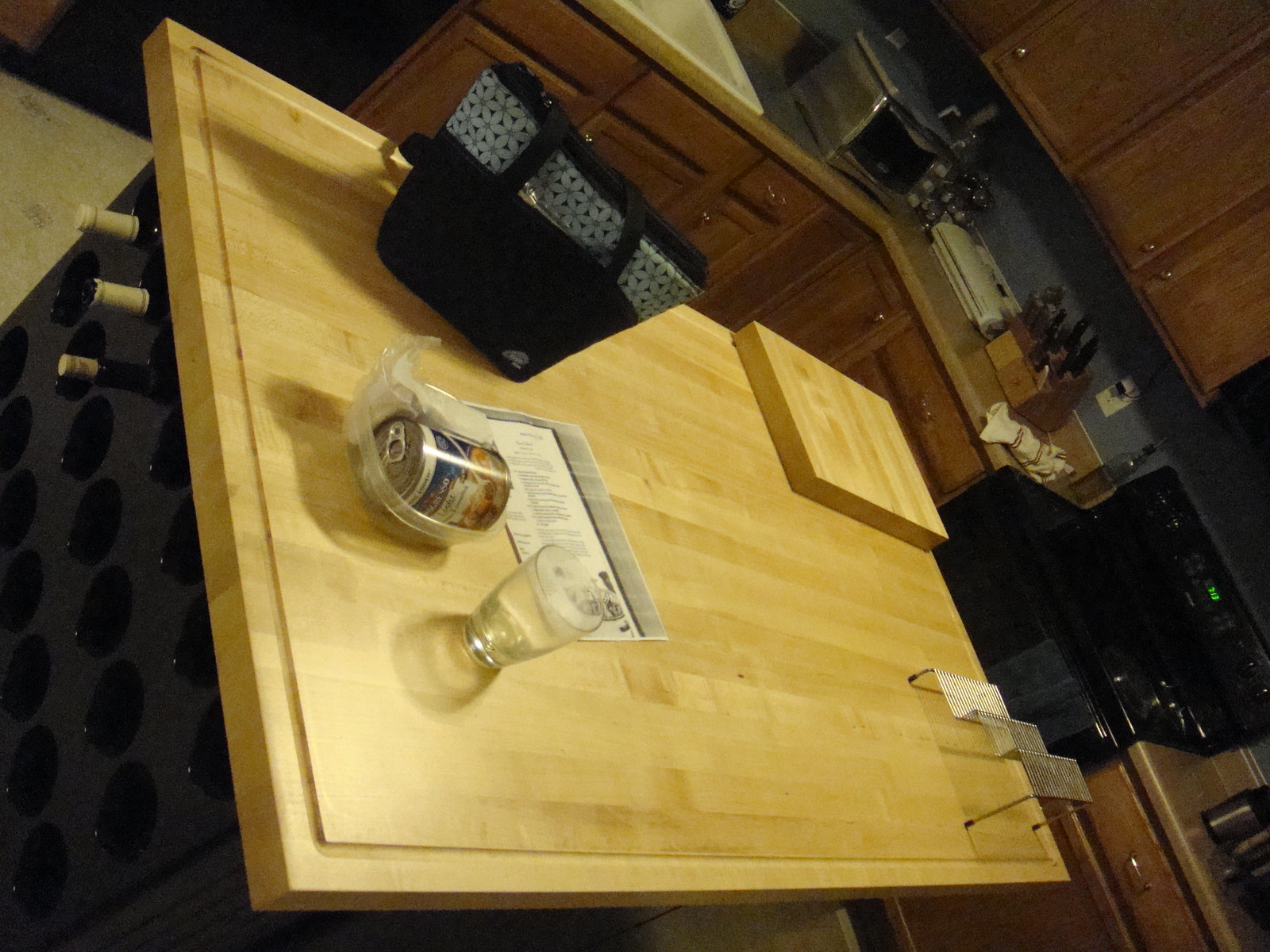The color snapshot captures a uniquely angled view of a 1970s-style kitchen, dominated by a wooden kitchen island featuring wine storage underneath. The photograph is taken from a slightly elevated position, creating an unusual perspective where the entire scene appears rotated. The horizon line is dramatically tilted, making the kitchen countertop and table surfaces appear almost vertical, around 70 degrees, adding a disorienting twist to the composition.

The kitchen exudes a vintage charm with its deep brown, maple wooden cabinets, contrasting against the paler oak finish of the kitchen island. Atop the island rests a distinctive handbag, adorned with a gray patterned band that suggests it might be a designer piece, possibly Yves Saint Laurent. This eccentric yet detailed composition offers a nostalgic glimpse into a 70s-era kitchen space, infused with a touch of modernity through the elegant accessory it holds.